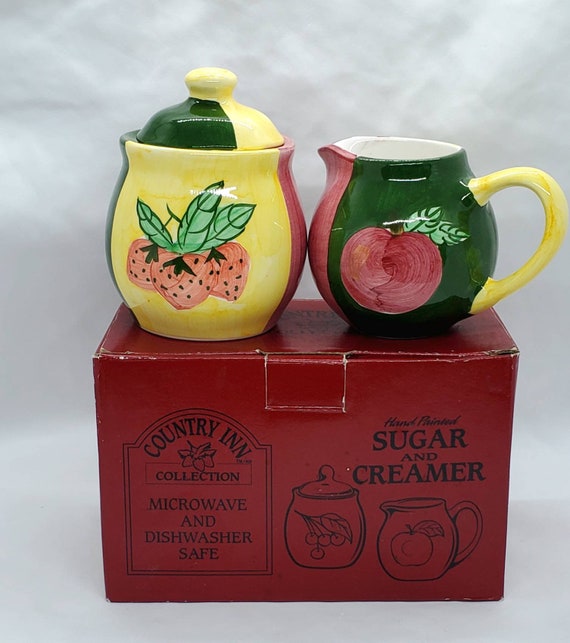This image features a set of ceramic sugar and creamer containers prominently displayed on top of a deep red box. The box, which appears to be part of the product's packaging, is labeled "Country Inn Collection" in black font and states that the items are microwave and dishwasher safe. On the left side of the box, there is also an illustration of the sugar and creamer set with the description "hand-painted sugar and creamer."

The sugar container, positioned on the left, has a yellow body adorned with painted strawberries and green leaves, and its lid is a combination of green and yellow. Meanwhile, the creamer, situated on the right, features a predominantly green body decorated with a painted red apple. Its handle is yellow, and there's a touch of red at the spout. The background of the image is a neutral gray and white, emphasizing the ornate and somewhat rustic aesthetic of the ceramics, which evoke a country farmhouse style.